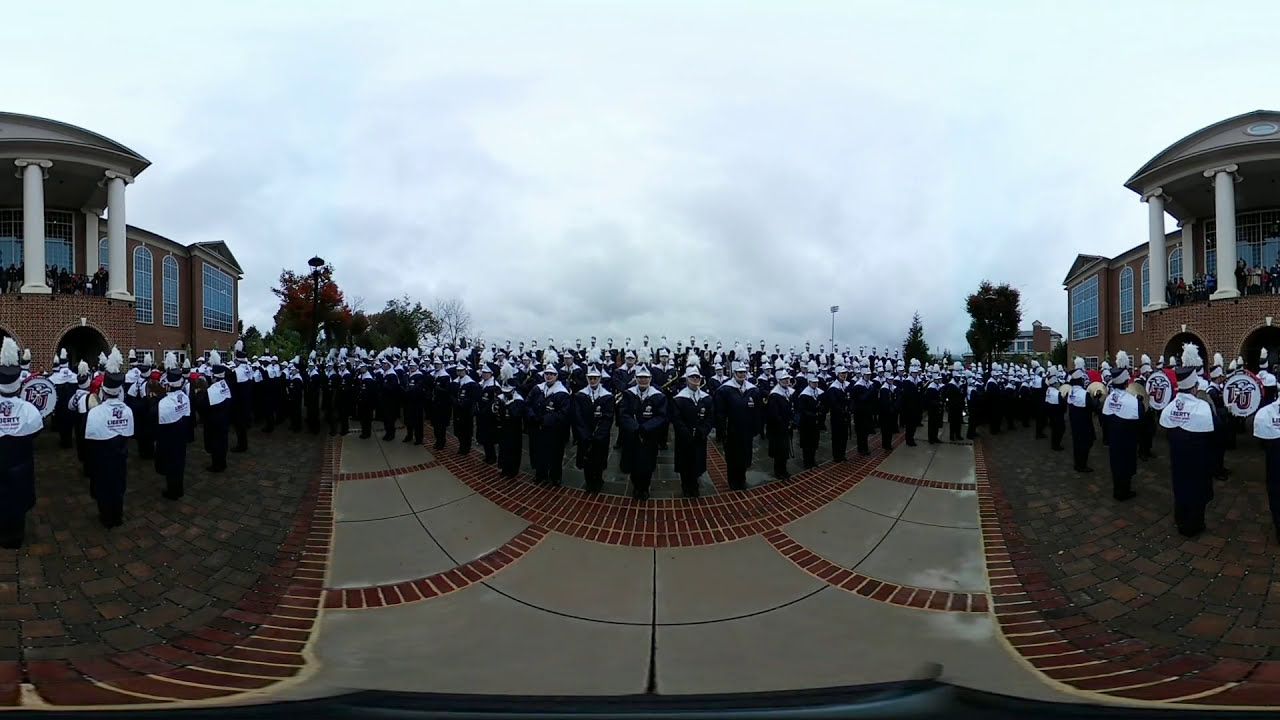This photograph, taken on a very overcast day with no visible blue sky, captures a university marching band preparing for a performance. The wide-angle, fisheye lens creates a mirrored, 360-degree effect, causing the buildings with tall, white pillar columns on the left and right sides to appear duplicated. The scene is well-illuminated despite the cloudy weather.

The band members, dressed uniformly in black pants and long-sleeved jackets with white helmets and collars, stand in formation on a stone tile pathway bordered by red bricks. The arrangement of the band resembles a central body with two wings fanning out to the sides. The drum lines are positioned on both the left and right, while the horn and woodwind sections hold their instruments at the ready in the center. The image suggests the presence of around 100 band members, poised for their march on this mirrored collegiate landscape, enlivened by nearby trees.